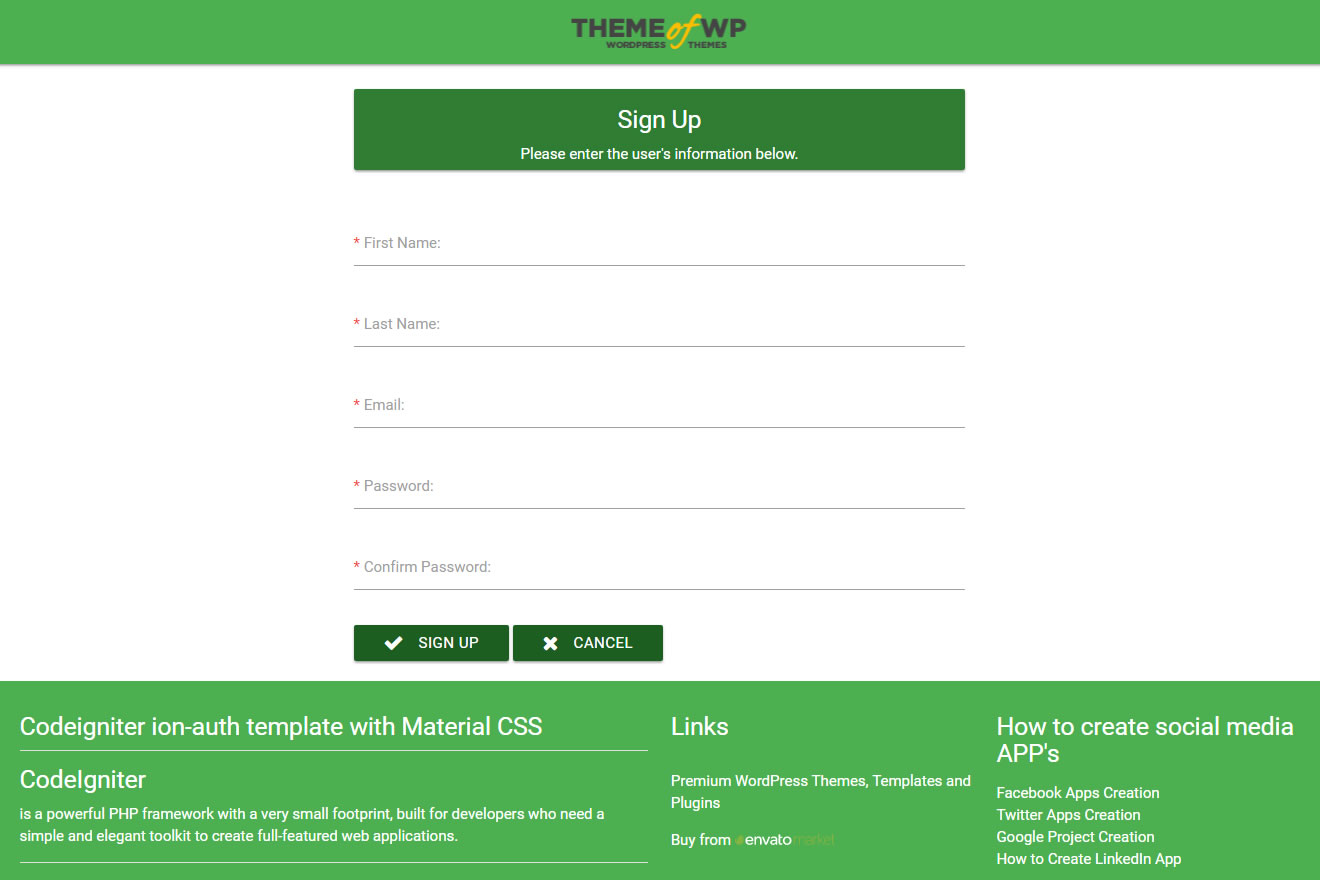**Screenshot Description:**

The screenshot features a WordPress theme with a predominantly green and black color scheme. 

- **Header Bar:** At the top, there's a vibrant green header bar centered with black text reading "Theme of WP." The word "of" stands out in an orange, handwritten script style. Below this, "WordPress Themes" is written in small capital black letters.

- **Sign-Up Overlay:** In the center of the main white field, there is an overlay sign-up area with a narrower, darker green header stating "Sign Up" in white text. Below this header, an instruction reads: "Please enter user information below." 

  - The form consists of five mandatory fields marked with asterisks:
    1. First Name
    2. Last Name
    3. Email
    4. Password
    5. Confirm Password

  - For each field, the label is in small text to the left of the corresponding field.

- **Action Buttons:** At the bottom of the sign-up form are two green buttons with white text:
  - The left button, marked with a check mark, reads "Sign Up."
  - The right button, accompanied by an 'x', reads "Cancel."

- **Footer Information:** The footer contains detailed text about the "CodeIgniter Ion-Auth Template with Material CSS":
  - "CodeIgniter is a powerful PHP framework with a very small footprint, built for developers who need a simple and elegant toolkit to create full-featured websites."

- **Footer Links and Text Alignment:**
  - To the right of center, it reads "Links:
    - Premium WordPress Themes
    - Templates and Plugins
    - Buy from Envato"
  - Further to the right is an option labeled "How to Create Social Media Apps," followed by four links:
    1. Facebook Apps Creation
    2. Twitter Creation
    3. Google Project Creation
    4. How to Create LinkedIn App